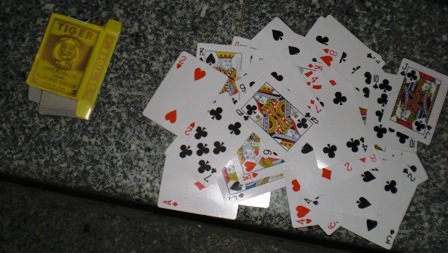In this rectangular, horizontal image taken from above, we observe a table or counter nearly filling the entire frame. The table features a polished black and gray marble design, and the dimly lit setting adds a moody atmosphere. On the upper left side of the table lies a worn, partially crushed box that once housed the playing cards scattered around. The box, opened on both ends, displays the word "Tiger" in brown print against a yellow background, with a spade symbol in the center and some blurred writing beneath it. The interior of the box is gray.

To the right of the box, a disarray of playing cards is strewn haphazardly, all facing up and forming a chaotic, messy circle. Notable cards visible in this tangle include the Two of Hearts, Seven of Clubs, King of Spades, Queen of Clubs, Jack of Spades, King of Hearts, Eight of Hearts, Four of Clubs, Ten of Clubs, Eight of Hearts, Two of Clubs, Jack of Clubs, and the Ace of Diamonds, among others. The King of Hearts and the Ace of Diamonds particularly stand out in the clutter.

The image is darker in the upper left corner, where shadows dominate, contrasting with the slightly lighter but still dim overall tone of the scene. On the lower left side, there appears to be an area beneath the table or an additional level of a darker surface, possibly a black floor or a secondary tabletop, contributing to the depth and texture of the image.